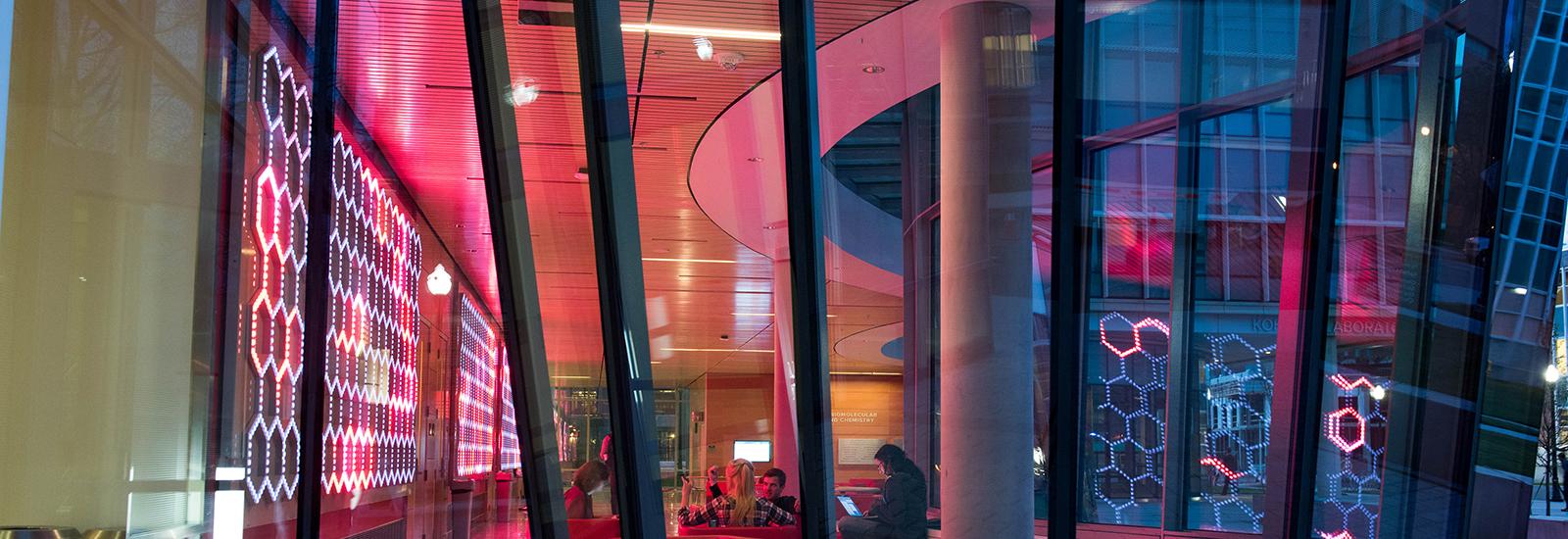This photograph captures the view through the large glass window of a tall, impressive Art Deco restaurant with modern architectural influences. The window is divided into five uneven sections with black and bluish separators. Inside, neon lights in shades of pink and purple cast a warm, vibrant hue across the room. The lighting highlights a striking geometric wall adorned with interconnected hexagons, arranged in rows and columns.

In the center of the image, a woman with a blonde ponytail, wearing a plaid shirt, is seen working at a laptop beside a column. To her right, a man is either reading a book or using his phone. Their table is cluttered with items, possibly food and drinks. Another two women are also present: one on the far left and one on the far right, each engrossed in their screens with their faces illuminated by the devices.

In the background, the letters "biomolecular" and "chemistry" appear on a wall, hinting that this might be a scientific establishment, perhaps a school or laboratory. The architectural design includes an exterior window with a curved style, through which one can catch glimpses of the word "laboratory" and partial letters "K-O" or potentially "R" or "B", reinforcing the scientific ambiance. Reflections on the glass add an ambiguous layer, blending the interior and exterior worlds.